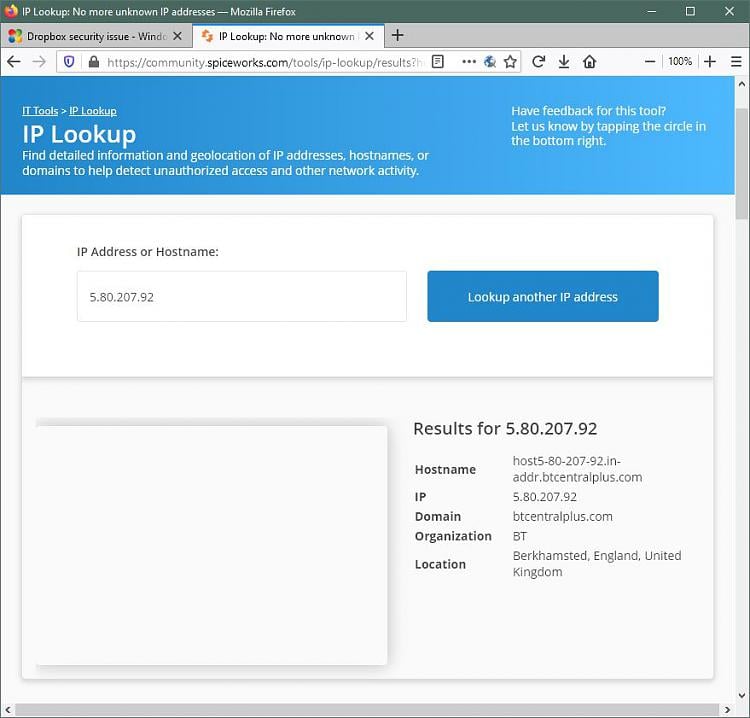Certainly! Here's a cleaned-up and detailed caption for the image:

---

In the image, a Mozilla Firefox web browser window is displayed with two open tabs. 

1. **Tab One**: The first tab, positioned on the left, is labeled "Security Issue" with a recognizable Windows icon featuring the four colors: red, blue, yellow, and green.

2. **Tab Two**: The second tab, situated to the right, is named "IP Lookup". It displays a webpage from "spiceworks.com".

The web address bar shows the URL "spiceworks.com", and below this, the webpage's header area has a blue background with white text. The left side of the header reads:
"IT Tools IP Lookup. Find detailed information and geolocation of IP addresses, hostnames, or domains to help detect and authorize access and other network activity."

The right side of the header includes a prompt:
"Have feedback for this tool? Let us know by tapping the circle in the bottom right."

Below the header, the main page has a white background with black text. On the left side, there is a form labeled "IP address or hostname," where the IP address "5.80.0.79.2" is entered. Next to this input field on the right is a blue button with white text that says, "Look up another IP address."

At the bottom left of the page is an empty high square, while the bottom right below the input field displays the results of the lookup for the IP address "5.80.0.79.2":
- Hostname: btcentralplus.com
- IP: 5.80.0.79.2
- Domain: btcentralplus.com
- Organization: BT
- Location: Berkhamsted, England, United Kingdom

---